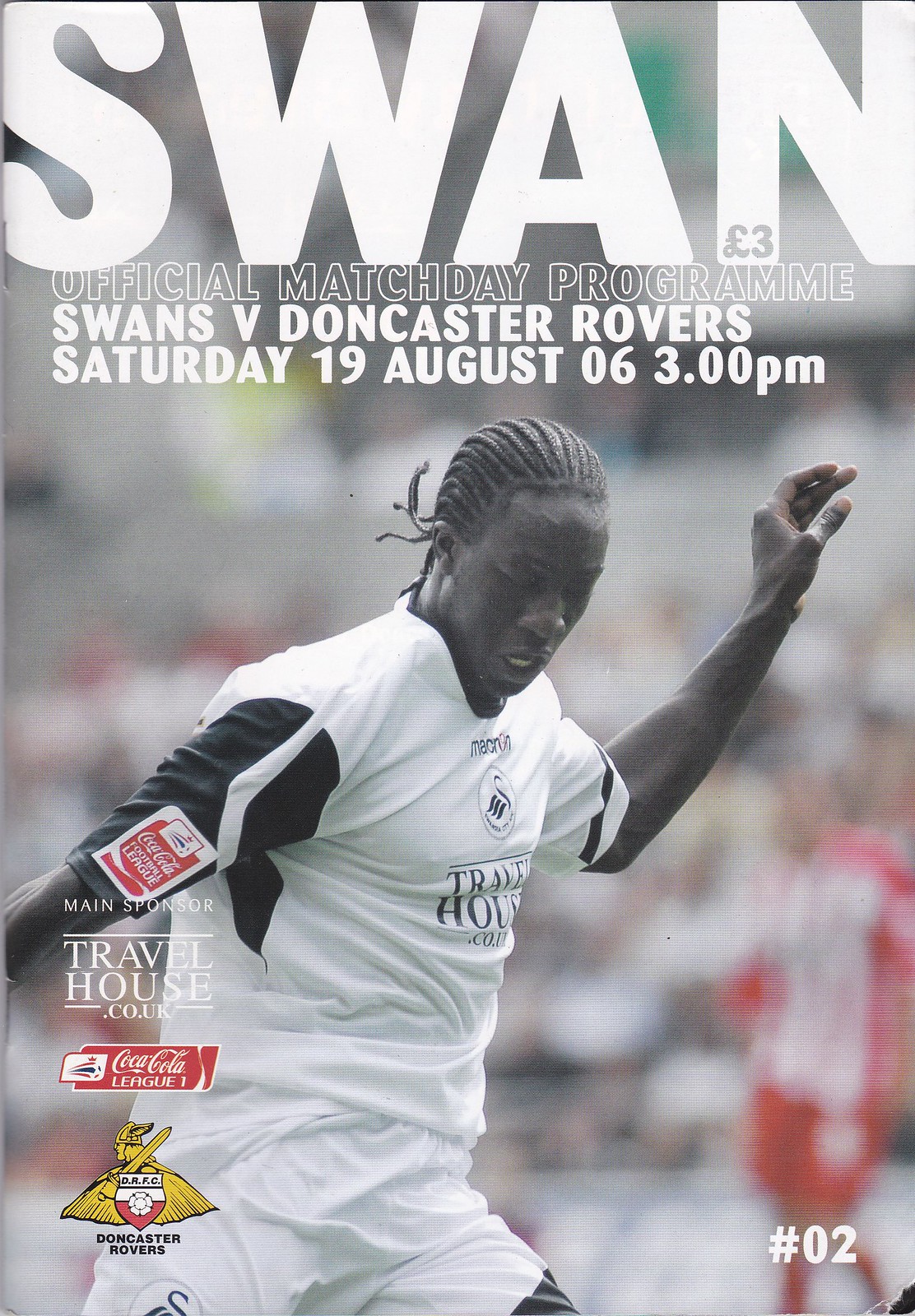The cover of the official matchday program, prominently labeled with the word "SWAN" in large, bold white letters at the top, features a detailed and striking design for the Swans vs. Doncaster Rovers game on Saturday, August 19 at 3:00 p.m. The subtitle beneath the main headline reads "Official Match Day Program." The central image captures a dynamic action shot of a black soccer player in a white uniform with black decorative elements on the sleeves. His left hand is extending towards the top right corner, and his hair flows behind him, indicating movement. The background is out of focus, with indistinct spectators in the stands and another player barely visible on the lower right. Along the lower left side, the program features advertisements, including the logo of the main sponsor, Travelhouse.co.uk, followed by Coca-Cola League and Doncaster Rovers, which includes an image of a Viking with a sword. The color palette of the cover includes black, brown, chocolate brown, white, red, goldish yellow, green, and gray. Notably, the program is marked with "Issue No. 02" at the bottom right corner, next to a small tear, and indicates a price of three euros.